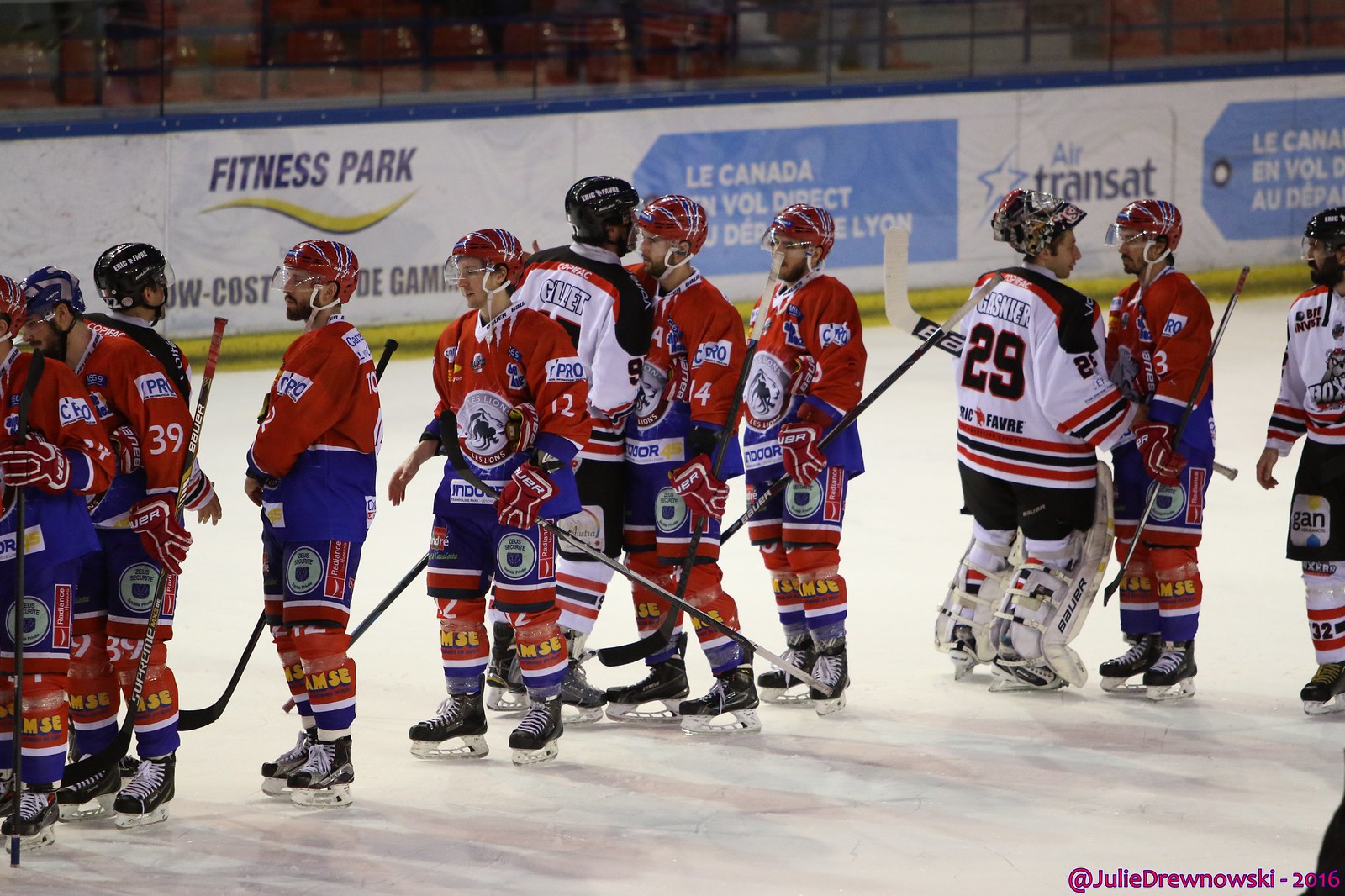In this photo taken by Julie Dronowski in 2016, two hockey teams are lined up on the ice, exchanging post-game congratulations. The rink serves as the backdrop with advertisements visible on the boards, including those for Fitness Park, Le Canada, and Air Transat. Eight players wearing red jerseys with blue accents, red helmets, blue shorts, and striped red and blue socks stand out prominently. Their opponents, clad in predominantly white jerseys with red, white, and blue stripes, dark shorts, and matching socks, include a player with the number 29 and the name Gassner on his back. Both teams are holding their sticks, facing each other in a line. The rink appears to be empty with no visible audience, and a lattice structure can be seen above the boards to prevent pucks from flying into the stands. A purple copyright mark in the lower right corner credits the photographer, Julie Dronowski.